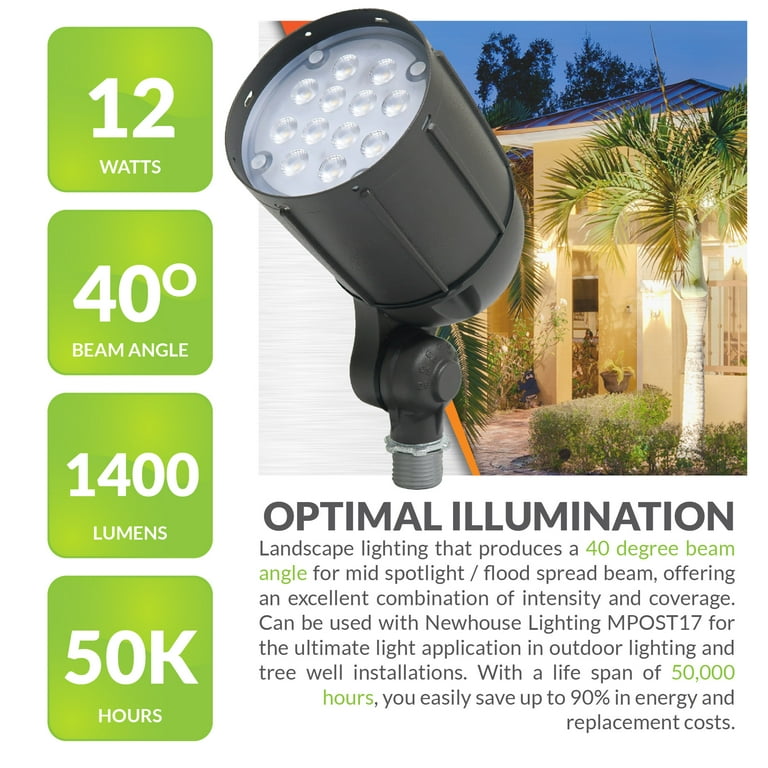This detailed advertisement showcases an outdoor light designed for optimal illumination and landscape lighting. Dominating the left-hand side, four striking green vertical boxes with white text highlight key specifications: 12 watts, 40-degree beam angle, 1400 lumens, and 50,000 hours of usage. To the right, a vivid color image features a large tan house bathed in light, with a black metal roof, pillars, palm tree, and surrounding greenery. Superimposed in front of this scene is the black light fixture, distinguished by its white lens dotted with LEDs, capable of swiveling for versatile installation. Below the vibrant visual, bold black letters proclaim "Optimal Illumination," followed by a detailed paragraph extolling the light's 40-degree beam angle, which delivers an excellent mix of intensity and coverage, making it ideal for outdoor and landscape applications, including new house lighting and tree well installations.